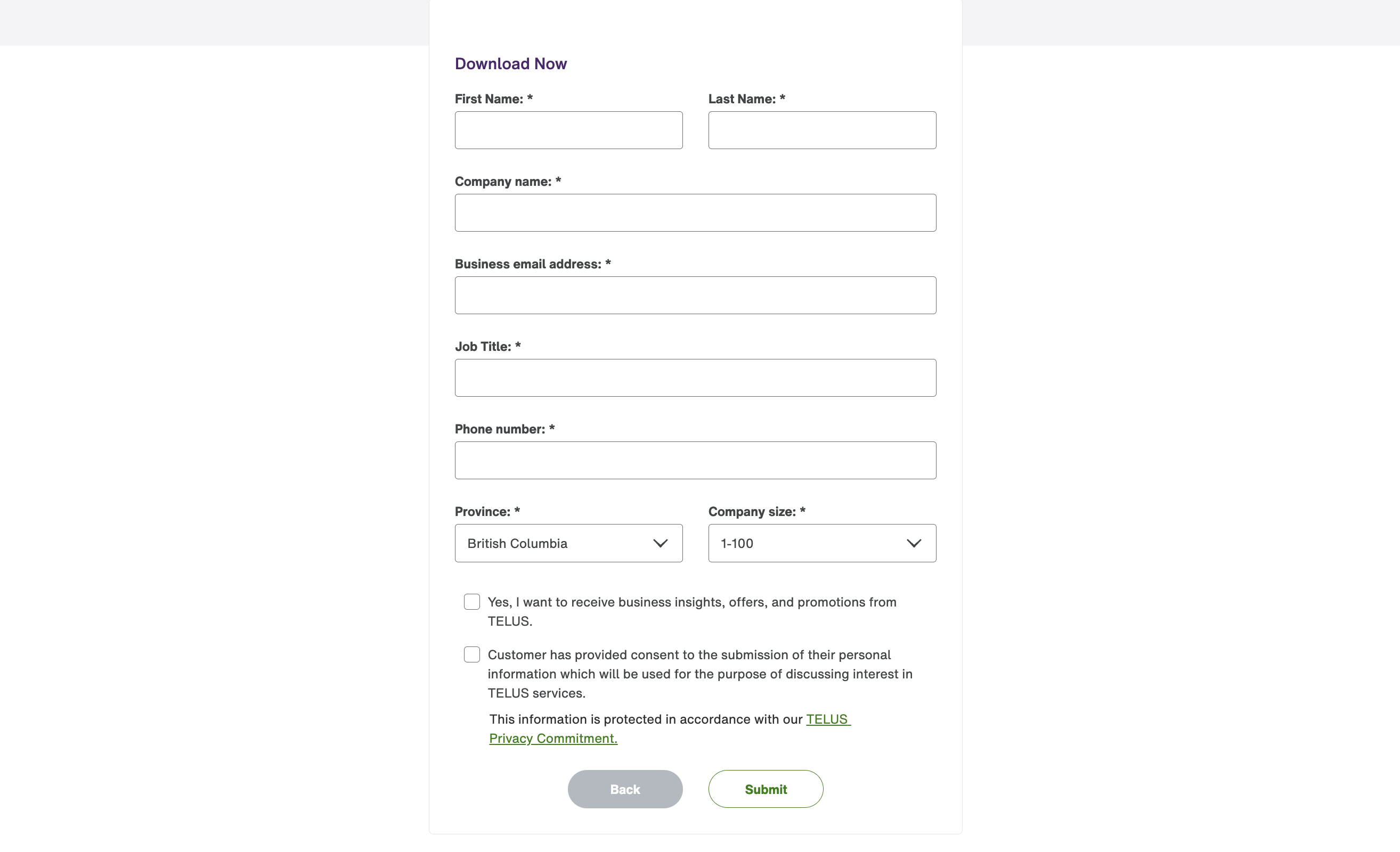In this screenshot of a website, the central section displays a form for downloading content. The layout features two empty panels on either side, topped with a light blue strip and filled with white below. The primary focus is on a white background in the middle, where the heading "Download Now" is prominently displayed in dark blue or purple font. Below this heading, various fields require user input:

- **First Name** (required) - The field is empty.
- **Last Name** (required) - The field is empty.
- **Company Name** (required) - The field is empty.
- **Business Email Address** (required) - The field is empty.
- **Job Title** (required) - The field is empty.
- **Phone Number** (required) - The field is empty.
- **Province** - A dropdown menu displays "British Columbia" as the selected option.
- **Company Size** - A dropdown menu shows "1-100 Employees" as the selected option.

Below these fields, there are two checkboxes:
1. The first checkbox, labeled "Yes, I want to receive business insights, offers, and promotions from TELUS," is not checked.
2. The second checkbox, labeled "Customer has provided consent to the submission of their personal information solely for the purpose of discussing interest in TELUS services," is checked.

A message indicates that the user’s information will be protected in accordance with TELUS’s privacy commitment, linked via a green underline. At the bottom of the form, there is a greyed-out "Back" button and a white "Submit" button with green text.

The form emphasizes a secure and user-friendly experience, guiding the user through required fields and options, with an accessible link to TELUS’s privacy policy for further assurance.